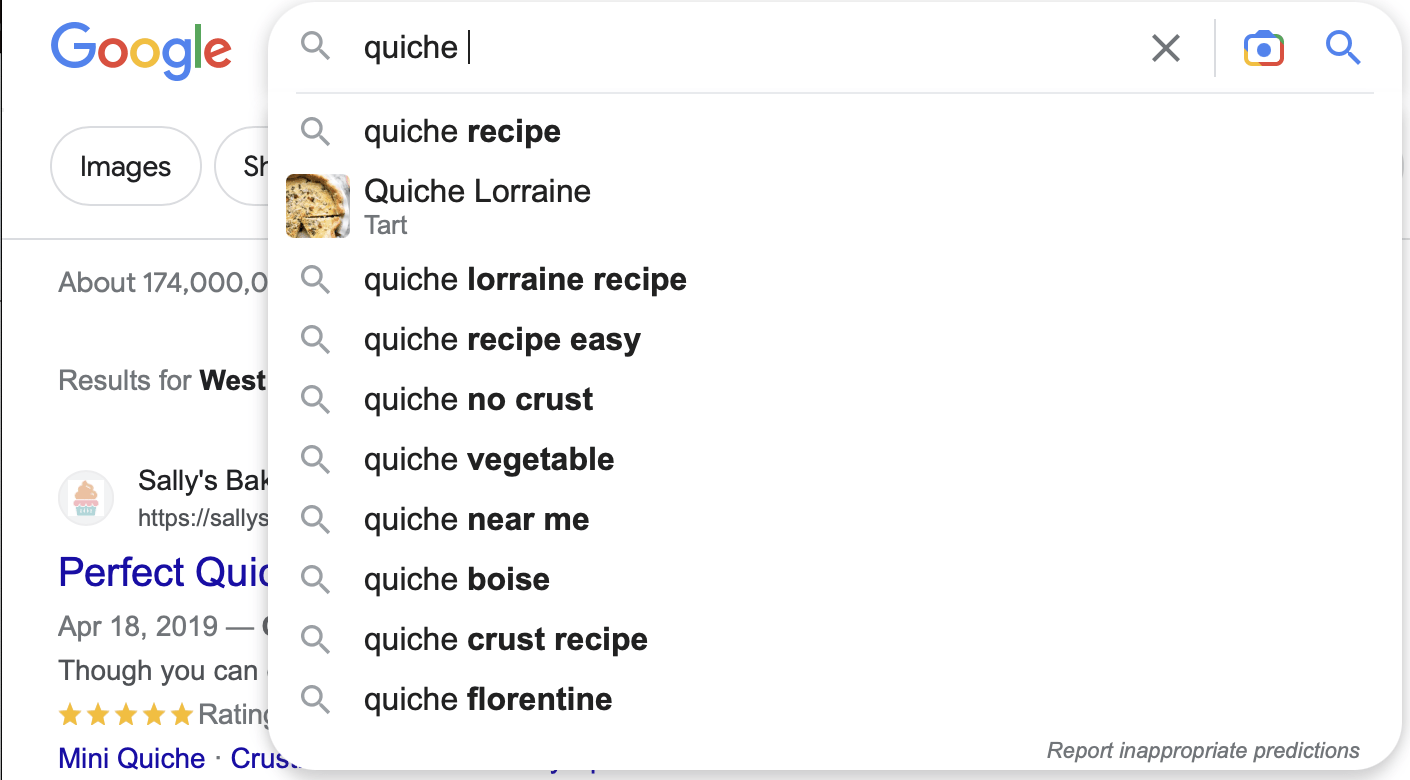This is a detailed screenshot from a Google search results page for the keyword "quiche." The search bar displays a dropdown menu with various search suggestions, each beginning with "quiche," followed by additional bolded keywords. The suggestions listed are:

1. Quiche recipe
2. Quiche Lorraine tart
3. Quiche Lorraine recipe
4. Quiche recipe easy
5. Quiche no crust
6. Quiche vegetable
7. Quiche near me Boise
8. Quiche crust recipe
9. Quiche Florentine

Each suggestion is preceded by a magnifying glass icon on its left side. At the top-right corner, there is italicized text stating "Report inappropriate predictions." 

In the background, the Google search page is partially visible. Below the Google logo, there is a "Images" bubble and further below, a segment of the search results is shown. The first search result is from "Sally's Bakery," dated April 18, 2019. The image associated with this result features a quiche dish, highlighting the various types of quiche recipes and options available.